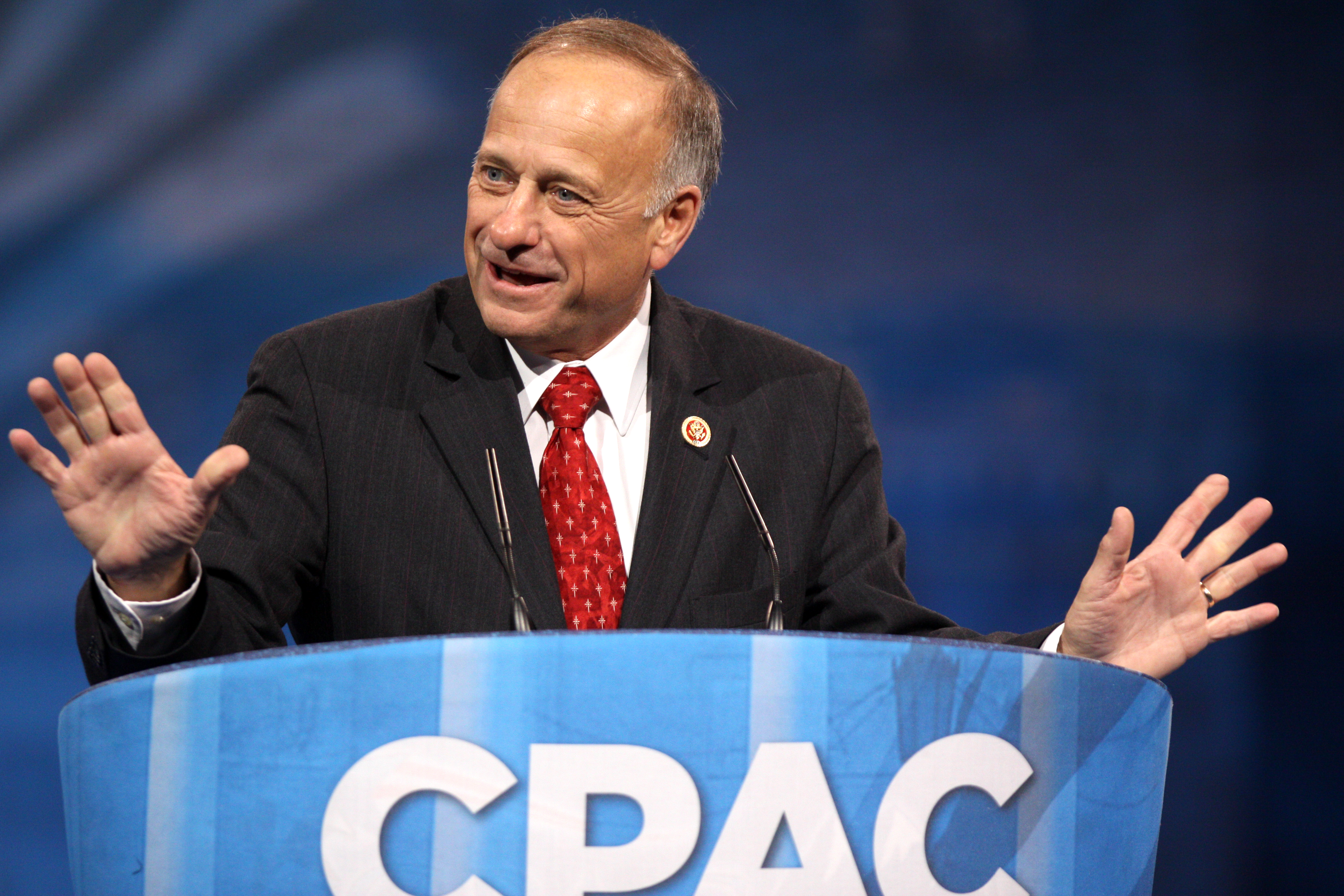In this detailed photograph taken indoors, an older gentleman, likely between 55 to 70 years old, is captured mid-speech at a podium. The podium, adorned in varying shades of blue with vertical stripes, prominently displays the letters CPAC in bold white capital letters. The man exudes an air of importance, dressed in a black pinstripe suit paired with a white dress shirt and a red tie adorned with gold designs, possibly crosses. A circular lapel pin further embellishes his attire. 

His hair, thinning and swept to the side, and his high forehead indicate his senior age. He has light skin, light blue eyes, and wears a wedding ring on his left hand. Speaking with great emphasis, he gestures widely, his palms visible and resting on the podium, which is equipped with high-tech microphones. The background is significantly blurred, a blend of darkish blue and gray hues, emphasizing his presence. With a slight smile, he looks towards the left side of the frame, engaging an unseen audience. The image, rectangular and about six inches wide by four inches tall, captures the moment with a sense of formality and gravitas typically associated with political action conferences like CPAC.